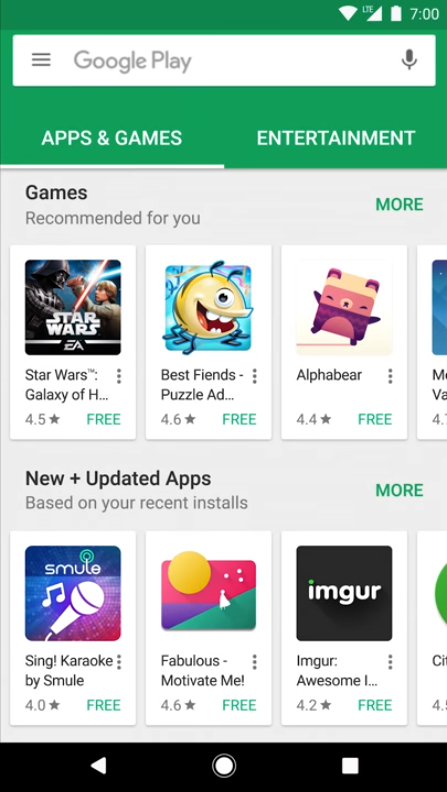The screenshot displays the Google Play Store interface, characterized by a medium green header at the top. Centered within the header is a white search bar that stands out against the green. On the left side of the search bar, three horizontally-stacked gray lines serve as a navigation menu icon, and to its right, the text "Google Play" is displayed in gray. Adjacent to this text on the far right of the search bar is a gray microphone icon.

Below the header, there are two selectable sections in white text: "Apps & Games" on the left and "Entertainment" on the right. "Apps & Games" is currently underlined in white, indicating it is the selected section. Directly below this selection, a medium gray background introduces the first category of content.

The first content row is labeled "Games, recommended for you," with a "More" option in green text to the right, inviting users to explore additional suggestions. Beneath this title, three game app selections are displayed, each housed within a white rectangle. The apps shown are:

1. "Star Wars Galaxy of Heroes" with a 4.5-star rating and listed as free.
2. "Best Friends Puzzle Adventure" with a 4.6-star rating and also free.
3. "AlphaBear" with a 4.4-star rating and free.

Following this, the next row is labeled "New & Updated Apps, based on your recent installs," similarly featuring a "More" option to the right. This row presents another trio of apps, also each within white rectangles:

1. "Sing! Karaoke by Smule" which holds a 4.0-star rating and is free.
2. "Fabulous - Motivate Me" with a 4.6-star rating and free.
3. "Imgur: Awesome Images & GIFs" with a 4.2-star rating and free.

At the bottom of the screenshot, a black rectangle contains three white icons, adding to the navigational features of the Google Play Store interface.